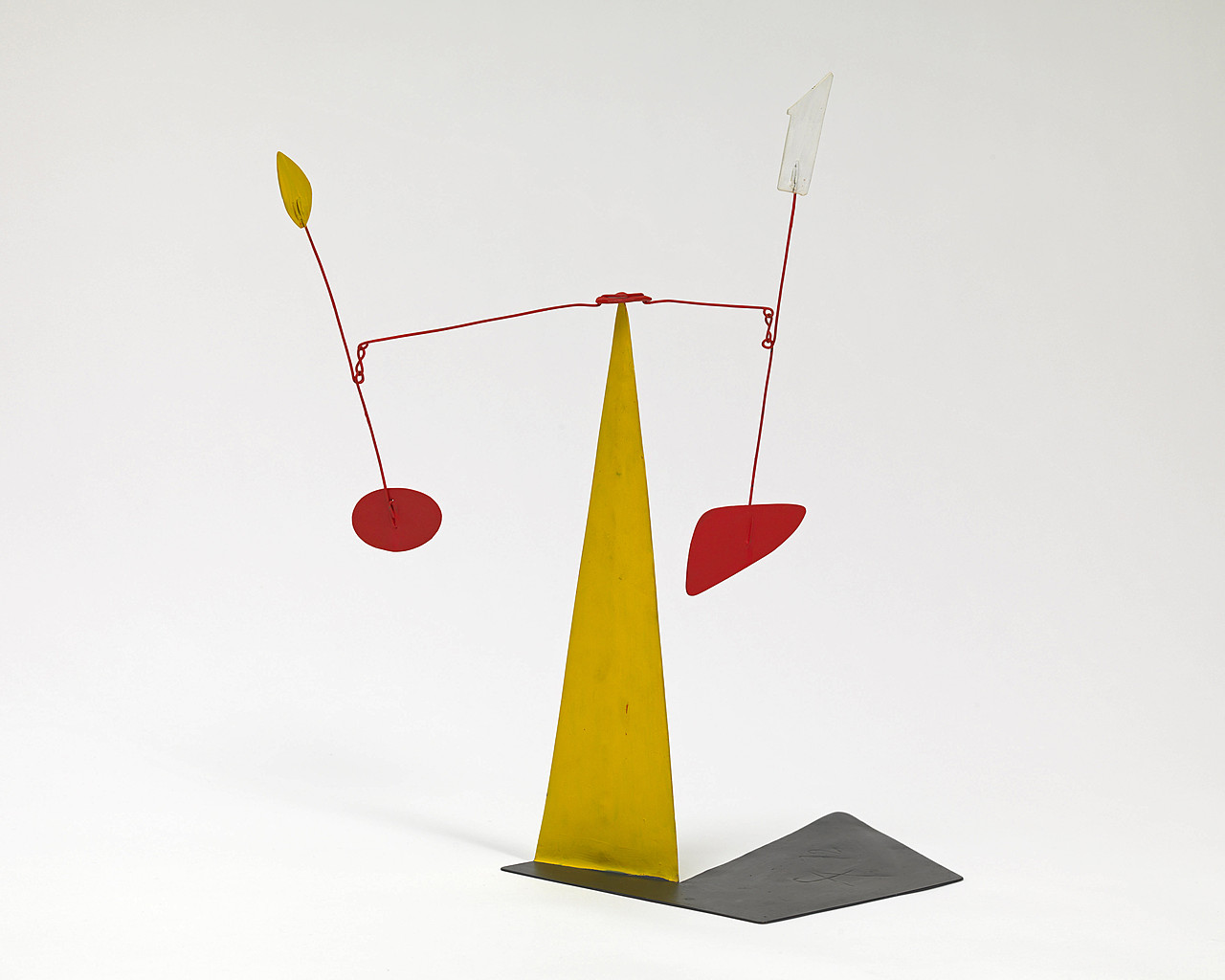The image showcases an abstract piece of art resembling a mobile, set against a light gray background that transitions to a white surface at the bottom. A dark gray, metal-like, flat structure shaped somewhat like the head of a golf club lies flat on the white surface, anchoring the composition. Extending from this base is a prominent yellow triangle, its right side blending into the background. At the apex of the triangle, two red wires stretch out horizontally, evoking the image of a balanced scale or a mobile.

To the right, a red wire extends upward and downward, connecting a small white rectangular shape at the top and an irregularly shaped red piece at the bottom. Another red wire branches to the left and down slightly, leading to additional wires that extend in various directions. These wires support an assortment of shapes, including a yellow irregular oval, a red circle, and other colorful forms.

The elements are delicately balanced, creating a sense of floating movement. The overall effect is a complex, harmonious arrangement of geometrical shapes and lines, all seemingly suspended in mid-air.